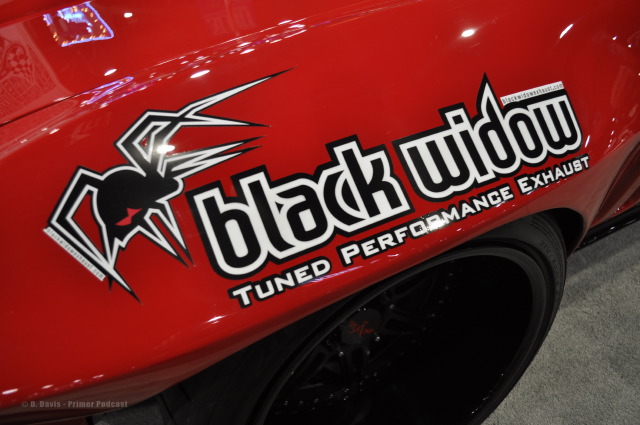This close-up image captures a high-gloss cherry red sports car, prominently featuring a bold decal. The focal point of the decal is a striking black widow spider illustration, characterized by its black body with a signature red hourglass marking, all outlined in white. Beneath the spider, the text "Black Widow" is displayed in large black letters with white borders, followed by the phrase "Tuned Performance Exhaust" in a similar style. The car's body curves gracefully around a black tire with a sleek five-spoke racing rim, which sits against what appears to be a gray, stone-like surface, possibly a garage floor. The image is tightly framed, revealing little of the car beyond the decal, tire, and a small section of the red back panel, all emphasizing the vehicle's modern and polished aesthetic.